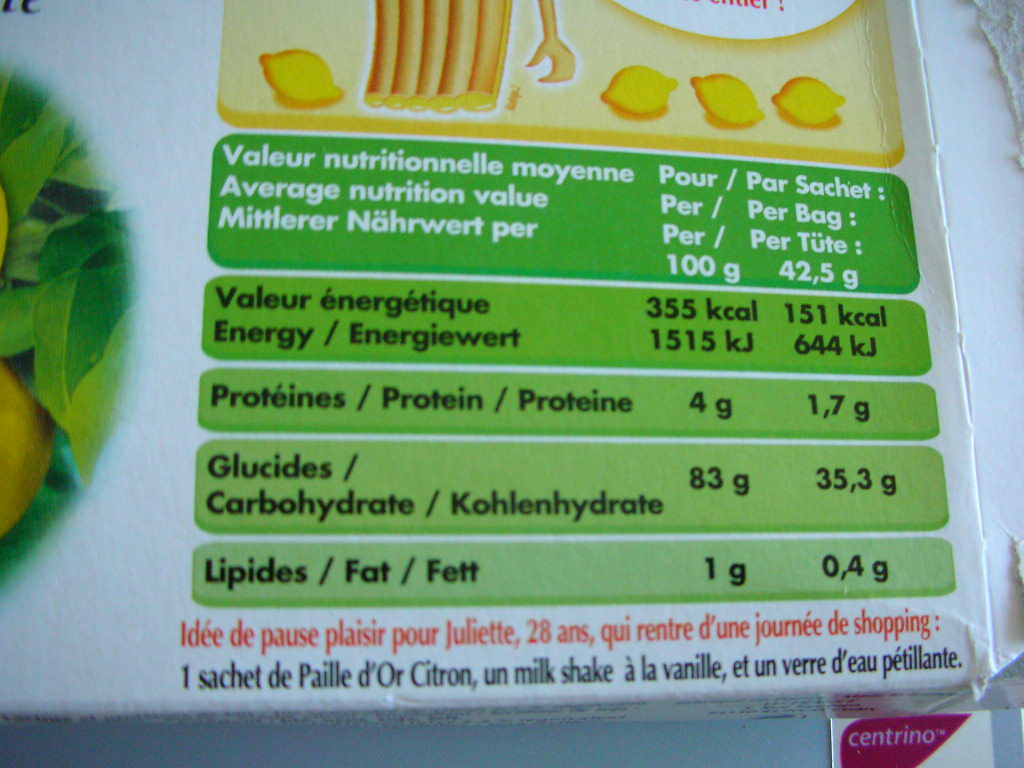This image showcases French packaging, likely from a food product, primarily displaying a nutrition label. The label is positioned on a white cardboard box. On the left-hand side of the box, part of a vibrant yellow lemon with green leaves is visible, gradually fading into the white background, adding a subtle, fresh aesthetic.

The top portion of the label features a yellow box with rounded edges containing the image of four yellow lemons. Additionally, there is a visual of several lemon-shaped cylinders clustered together with a hand extending from the group, adding an artistic touch.

Below the vibrant yellow box, a green-colored section reads "Tableau Nutritionnel Moyen," which translates to "Average Nutritional Value." The label continues to provide nutritional details, including energy content, listed as "1,515 kilojoules." Following this, it presents information on protein, carbohydrates (glucides), and fats (lipids), each category placed in progressively lighter shades of green boxes as the list descends, ensuring a clear and structured presentation of the nutritional information.